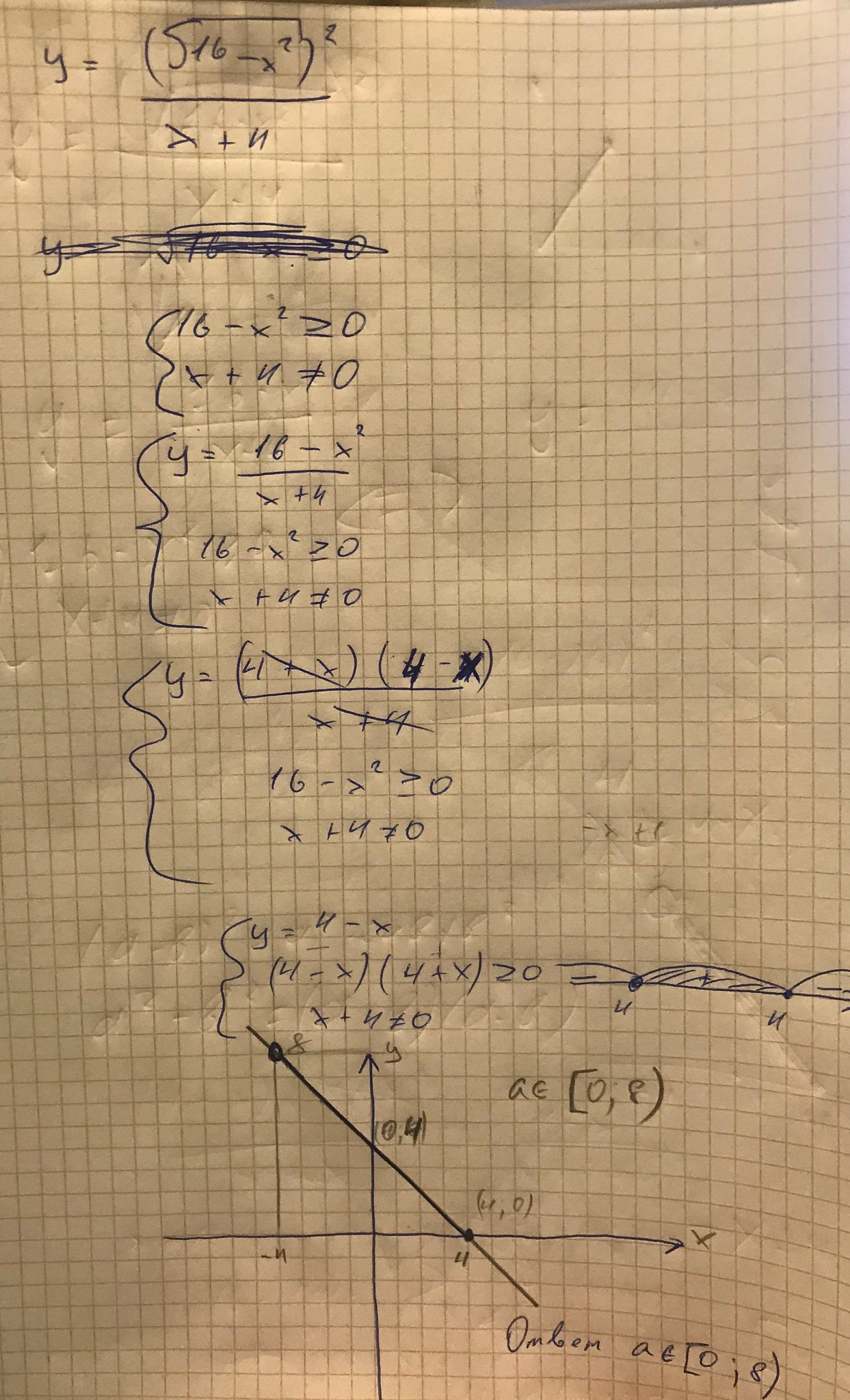This image features a piece of graph paper densely covered with handwritten mathematical notations. The handwriting, executed in a blue ballpoint pen, appears markedly sloppy and heavily indented into the paper due to significant pressure exerted by the writer.

At the top of the sheet, the equation "y = (5^16 - x^2)" is written, with the exponents and variables appearing somewhat jumbled. Below this, another equation starting with "y" has been scratched out multiple times, creating a chaotic visual effect. This is followed by a sequence of mathematical expressions and inequalities:

- "(16 - x^2) < 0"
- "y + u// ≠ 0"
- "(16 - x^2) / (x + 4)"
- "16 - x^2 <= 0"
- "x + 4 = 0"
- "(y^4 + x^4 - x(x + 4))"

Beneath these formulas, there is a hastily drawn graph displaying the x and y axes, with several points plotted on it. The combination of the inconsistent handwriting and numerous corrections makes the document difficult to interpret. The graph at the bottom serves as an attempt to visualize some of the aforementioned equations or inequalities.